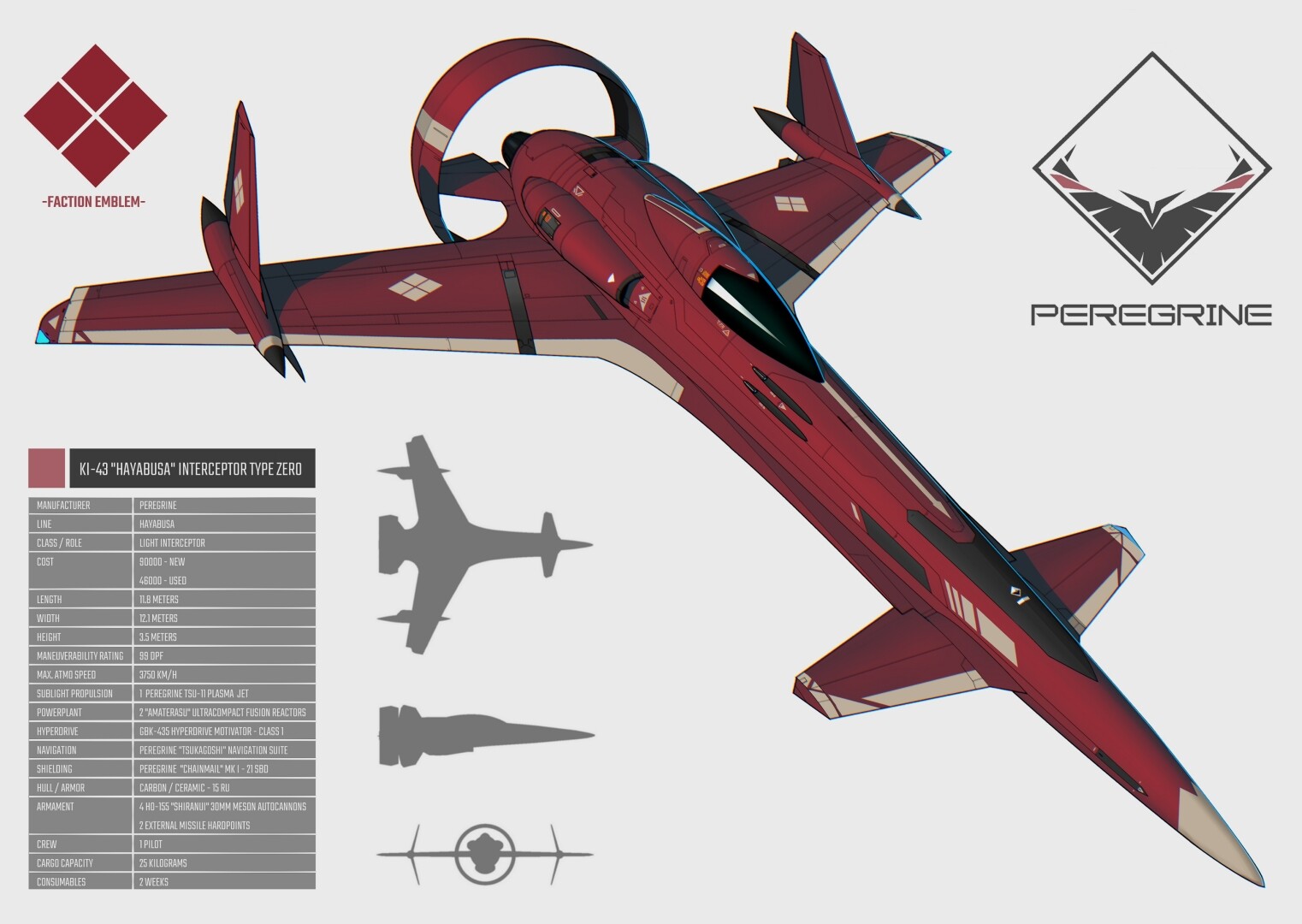The image features a detailed, artistic rendering of a futuristic fighter jet with a unique design, set against a black-gray background. The central plane is needle-like and predominantly red, featuring a distinctive pusher propeller at the rear. Notably, the smaller wings are positioned at the front, while the longer wings extend from the rear, breaking conventional aircraft design norms. The cockpit window is entirely black, offering a sleek, tinted appearance. 

In the upper left corner, there is a faction emblem formed by four red diamonds creating a larger diamond shape, labeled "Faction Emblem." This emblem also appears on the plane's rear wings. Below the main plane image, the bottom left corner includes detailed specs like length, width, height, speed, navigation, shielding, crew capacity, cargo specifications, cost, and manufacturer information, under the title "KI-43 Kuiper-0 Interceptor Type-0."

The upper right corner displays another emblem within a stylized gray diamond box, featuring an image of a falcon. Below this, "Peregrine" is written in dark gray letters. Additionally, there are gray silhouette images depicting different angles of the jet (including side, top, and front views) in the left-hand corner, providing a comprehensive view of its design. Light gray or tan markings are also present on the jet's front part, enhancing its detailed appearance.